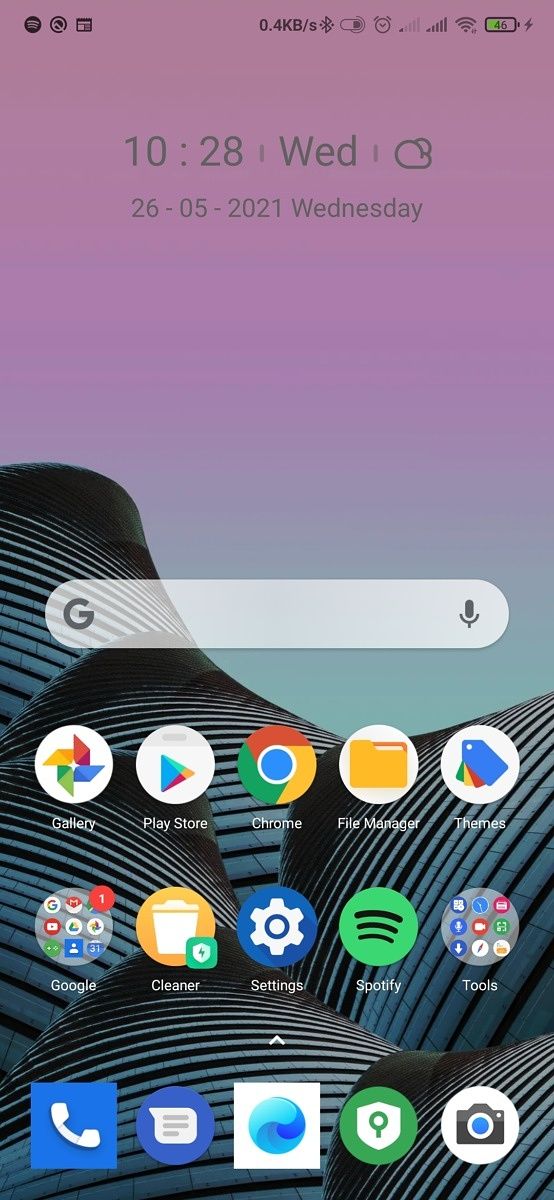In this image captured from the front screen of a cell phone, the display features a variety of prominent elements. At the very top, there are multiple icons on both the left and right sides of the screen. The date is displayed as "10/28," followed by "Wed," indicating Wednesday, and it shows a cloud icon representing weather conditions. The date is further clarified as "26-05-2021."

In the top right, a battery icon shows a green bar indicating a charge level of 46%, with a charging symbol next to it. The background of the screen transitions from a pinkish-purple hue at the top, gradually changing to a deeper purple, and eventually blending into teal and green towards the bottom.

The lower portion of the screen displays a hilly landscape composed of teal, green, and black tones. Centrally located, there is a search bar with a "G" on the left side, representing Google, followed by an empty field and a microphone icon on the right. At the very bottom of the screen, apps of various colors are arranged, ready for the user's selection.